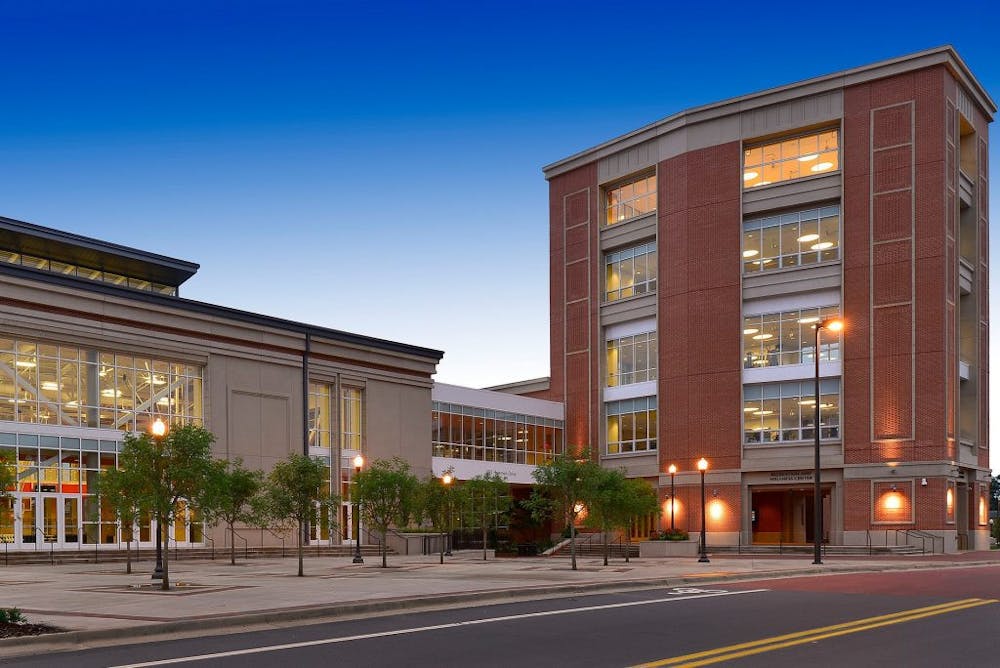The image captures a city street at dusk, with a road prominently featuring double yellow lines running down its center and a designated bike lane marked in white. On one side of the street is a spacious sidewalk that transitions into a broad plaza area, adorned with scattered young trees and numerous black street lamps topped with white lights. On the left side of the image, there's a two-story beige building with several ground-floor doors and a large glass window on the upper floor, framed in white. This building appears to connect via a white walkway to a taller adjacent structure made of red brick. This red brick building stands five stories tall, with vertical columns and multiple large glass windows on each floor. The sky above is a deepening blue, indicating either early morning or the approach of night, complemented by the clear, starless expanse, suggesting a serene urban setting.